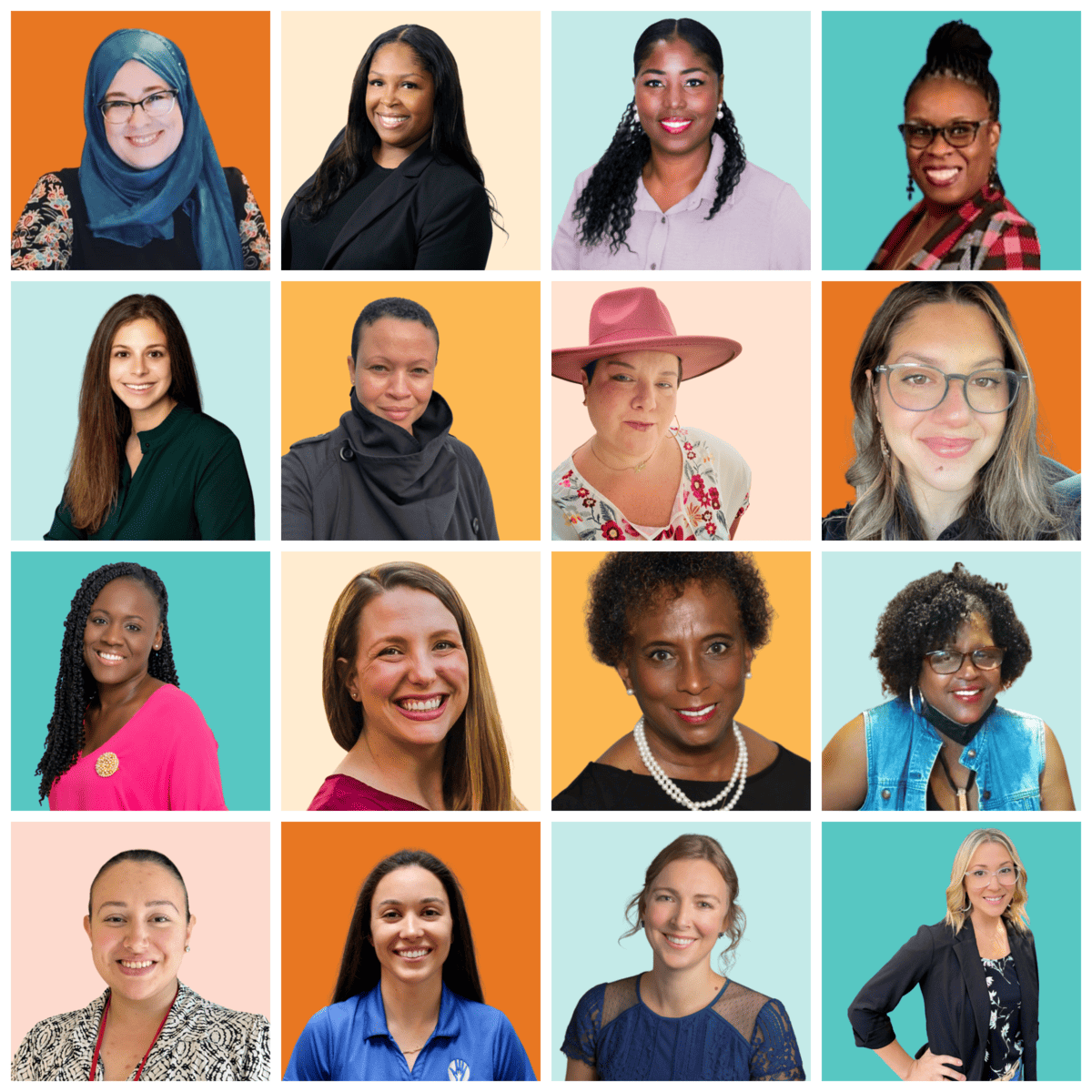The image is a grid of sixteen profile pictures, organized in four rows and four columns. Each picture features a woman against various backgrounds, capturing a diverse array of styles and expressions.

#### Top-Left Quadrant:
1. **First Woman:** Wearing glasses and a hijab, set against an orange background.
2. **Second Woman:** Dressed in a black shirt with a matching blazer.
3. **Third Woman:** Sporting a purple shirt and large earrings.
4. **Fourth Woman:** Wearing a plaid blazer with glasses and large earrings.

#### Second Row:
5. **Fifth Woman:** Clad in a black shirt.
6. **Sixth Woman:** Also in a black shirt but distinguished by a black cowl around her neck.
7. **Seventh Woman:** Dressed in a flowered shirt with a pink hat.
8. **Eighth Woman:** Wearing glasses.

#### Third Row:
9. **Ninth Woman:** In a pink shirt.
10. **Tenth Woman:** Wearing a red shirt.
11. **Eleventh Woman:** Dressed in a black shirt adorned with a pearl necklace.
12. **Twelfth Woman:** Sporting a denim vest.

#### Bottom-Right Quadrant:
13. **Thirteenth Woman:** Wearing a black and white blazer.
14. **Fourteenth Woman:** In a blue polo shirt.
15. **Fifteenth Woman:** Her hair is tied up, and she is dressed in a blue lace shirt.
16. **Sixteenth Woman:** Clad in a black blazer.

Each woman's unique style, from colorful attire to accessories like glasses and earrings, creates an engaging and vibrant collage.